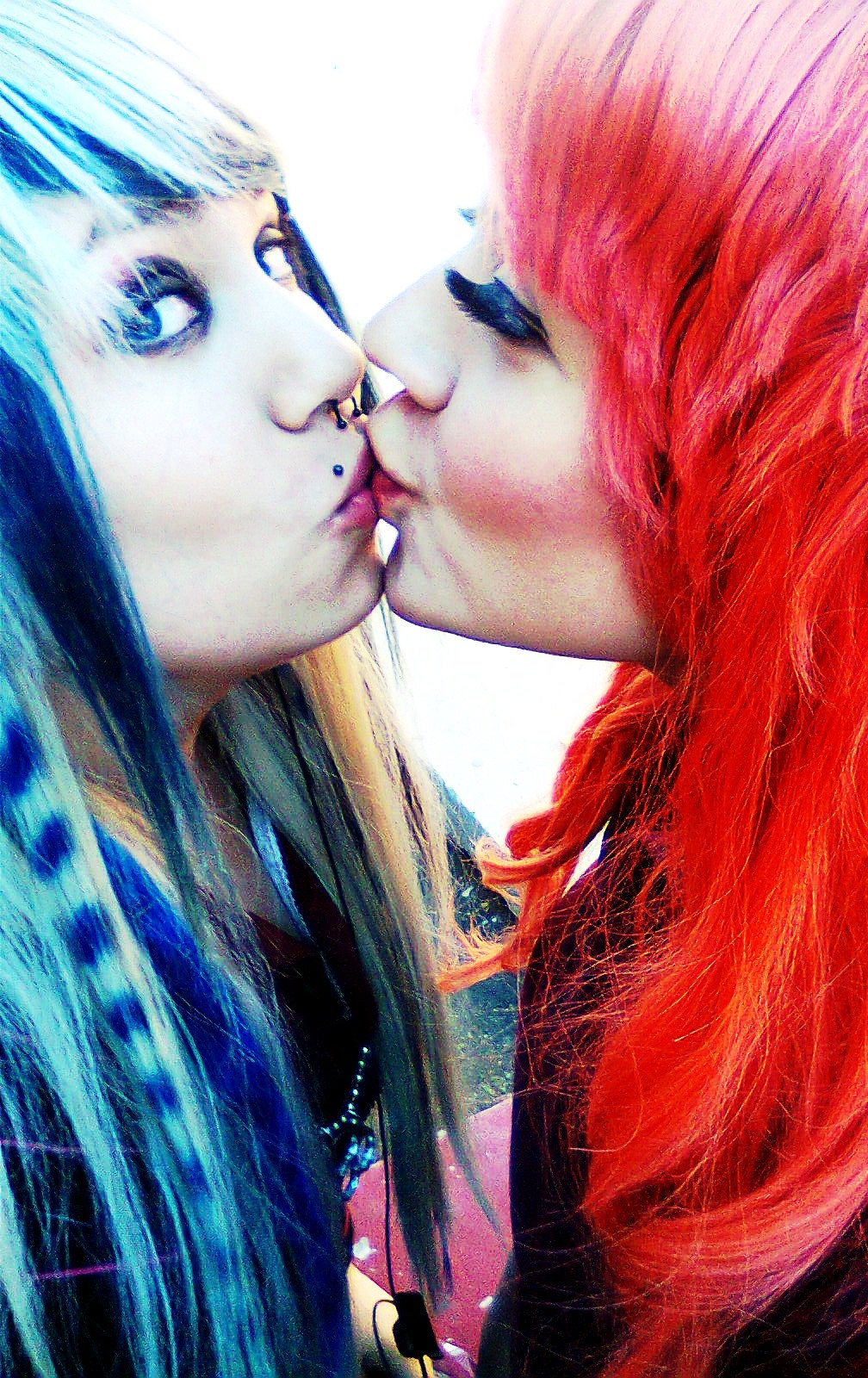This image portrays an intimate moment between two women, captured from their chests up. The woman on the left, with striking blue hair accented by lighter blue highlights and dark blue striping, sports a septum piercing and a piercing above her lip. Her blue eyes, accentuated by heavy blue eyeshadow and mascara, gaze directly at the camera with a slightly puzzled expression. She wears a black shirt and a blue gemstone necklace. The woman on the right, with long, richly hued red hair and excessively long, thick eyelashes, is seen in profile with her eyes either closed or heavily made up, obscuring them. She has pale skin, a touch of blush, and wears pinkish lipstick along with a black shirt. The background is a washed-out, light-colored wash, and together, the couple's vivid appearance and tender kiss stand out against this stark backdrop.